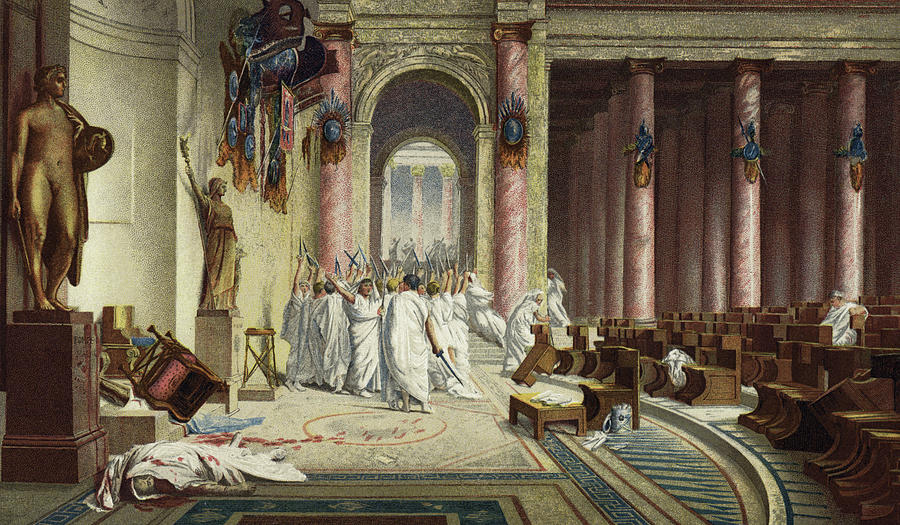The image depicts a highly detailed painting, exuding an old-fashioned, classical aura reminiscent of the Roman era. The scene is set within the grand interior of what appears to be a church or temple, defined by light brown or pink pillars with a marble texture and numerous wooden chairs, some of which are overturned.

At the heart of the composition is a chaotic and grim depiction of an assassination. A group of individuals, all clad in long, flowing white robes, are gathered centrally, their hands raised, brandishing weapons that resemble daggers, as if in a moment of frenzied chanting. 

In the immediate foreground lies the tragic focal point: a man, draped in a blood-stained white sheet, collapsed and lifeless. His right arm extends from under the sheet, his face partially obscured yet revealing closed eyes. Blood pools beneath his head, trailing down the steps upon which an overturned red chair also rests, signaling a previous struggle.

Flanking the macabre scene are bronze statues, further emphasizing the somber tone. The muted colors across the painting add to its chilling and historically evocative atmosphere.